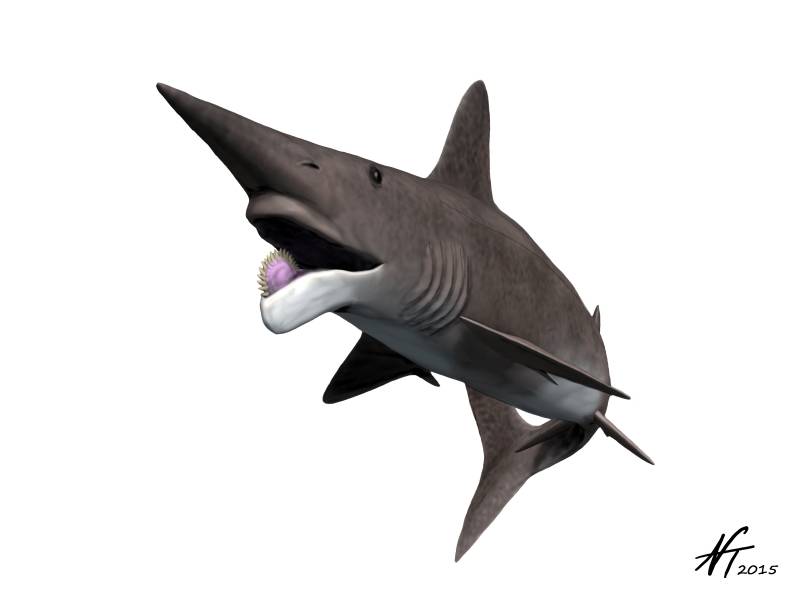The image depicts a detailed, digitally created rendering of a shark set against a plain white background. Viewed from its underside, the shark exhibits a dark, dull gray coloration on its upper body, with a lighter gray underside and a white lower jaw. The shark is angled with its tail fin positioned behind it, its body curving toward the right, and its head and open mouth directed to the left. Notably, the shark's mouth contains an unusual, saw-like protrusion reminiscent of a tongue with jagged teeth on it, adding a peculiar twist to its appearance. The shark also features a distinct, horn-like nose that is sharp and triangular. A small black eye is visible on its head. In the lower right corner of the image, the artist's initials "NT" and the date "2015" are inscribed in black cursive, serving as the artist's signature.